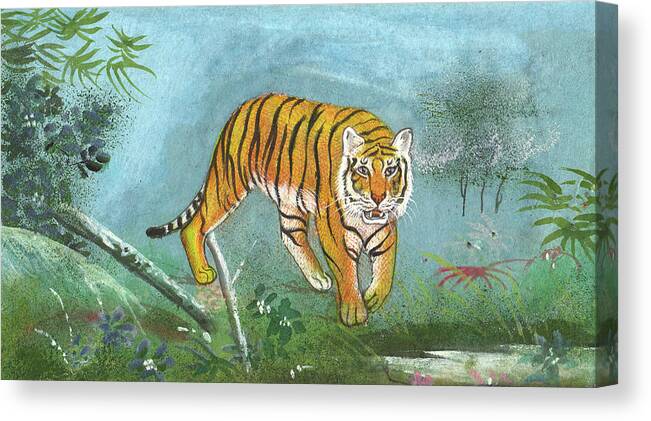In this detailed and vibrant hand-drawn mural, a majestic Bengal tiger dominates the canvas, wonderfully rendered in three dimensions. From a slight rightward angle, the image showcases the tiger's entire right side as it strides diagonally from the upper left to the lower right corner of the image. The tiger, with its classic yellowy-orange coat adorned with black vertical stripes, displays its white-furred underbelly and patches around its mouth and whiskers. Its vivid blue eyes, black pupils, upward-pointing ears, and slightly open mouth add a lifelike quality to its intense gaze at the viewer. The tiger’s right front paw is firmly on the ground, while the left is slightly raised, crossing over a gray tree branch or log, with its tail displaying alternating white and black bands, ending in a solid black tuft.

A lush, abstract jungle forms the backdrop, with varied green foliage extending across the scene. On the right, light green, red, and white foliage coexist with small trees above the tiger’s ear, while dark and lighter green shrubs populate the left edge. The sky behind blends shades of misty gray and blue, suggesting an early morning ambiance, accentuated by cloud-like mists around the bushes. In the foreground, subtle, arc-like hills or raised bushes emerge, leading to a shimmering water body in the bottom right corner which the tiger is approaching. The scene combines the serene beauty of nature with the powerful presence of the tiger, encapsulated within the curved edges of the canvas that blend seamlessly into the frame.